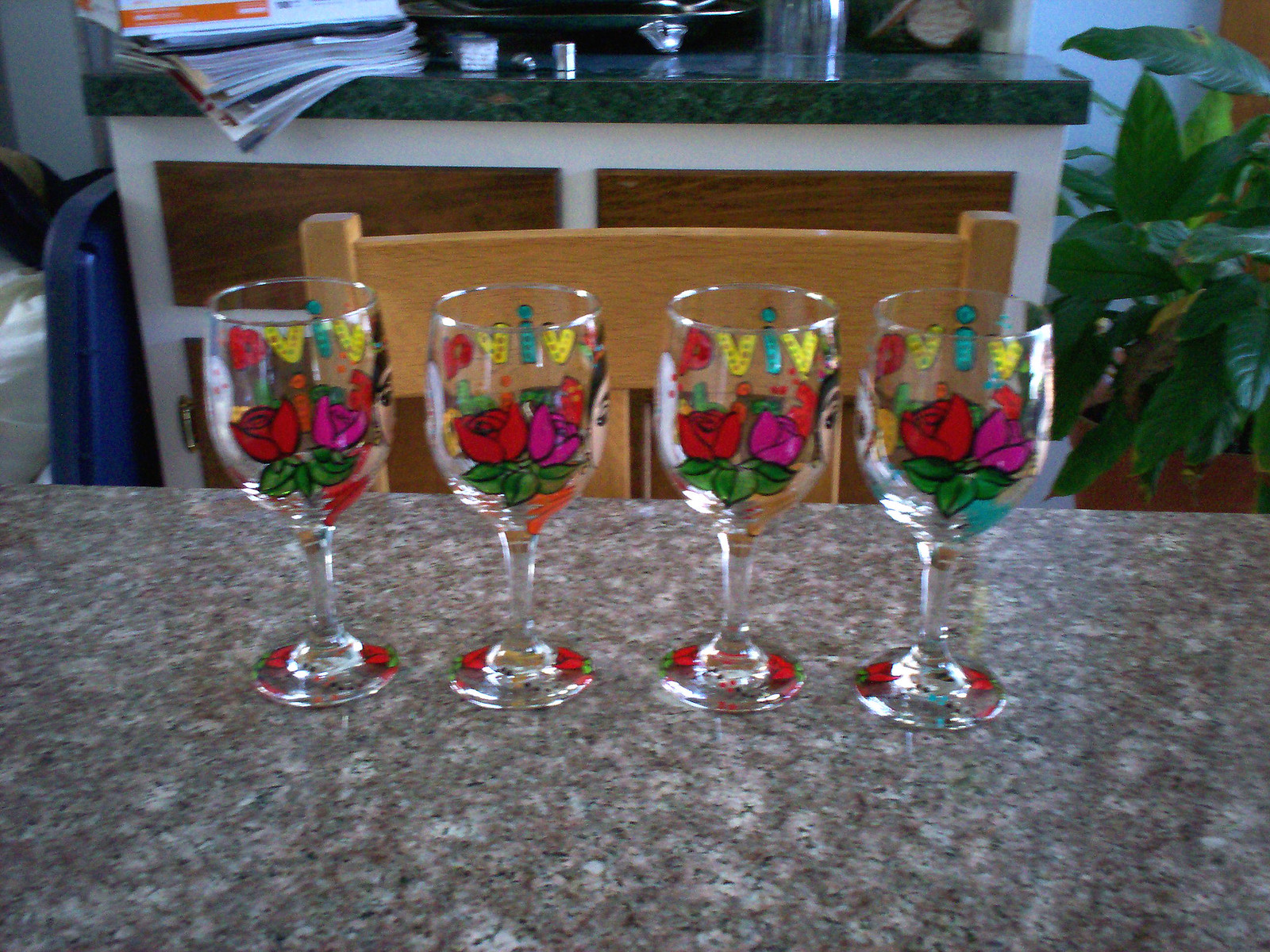This photograph captures a detailed scene in a kitchen. Central to the image are four clear stemmed wine glasses, each painted identically with vibrant floral designs featuring red and pink roses along with bright green leaves. The lettering on the glasses, which appears to spell "VIVA" in yellow, blue, and sometimes red lowercase letters, adds a festive touch. Additionally, the bases of all four glasses are adorned with red rose petals. These glasses rest on a gray and white marble-like countertop. In the background, a light brown wooden chair is positioned in front of a kitchen island equipped with brown drawers and a dark green granite or Formica top. To the right, a large rubber tree plant in a terracotta pot provides a touch of nature, while nearby, a chrome object and some magazines or papers can be seen on the back counter, hinting at the everyday life in the kitchen.